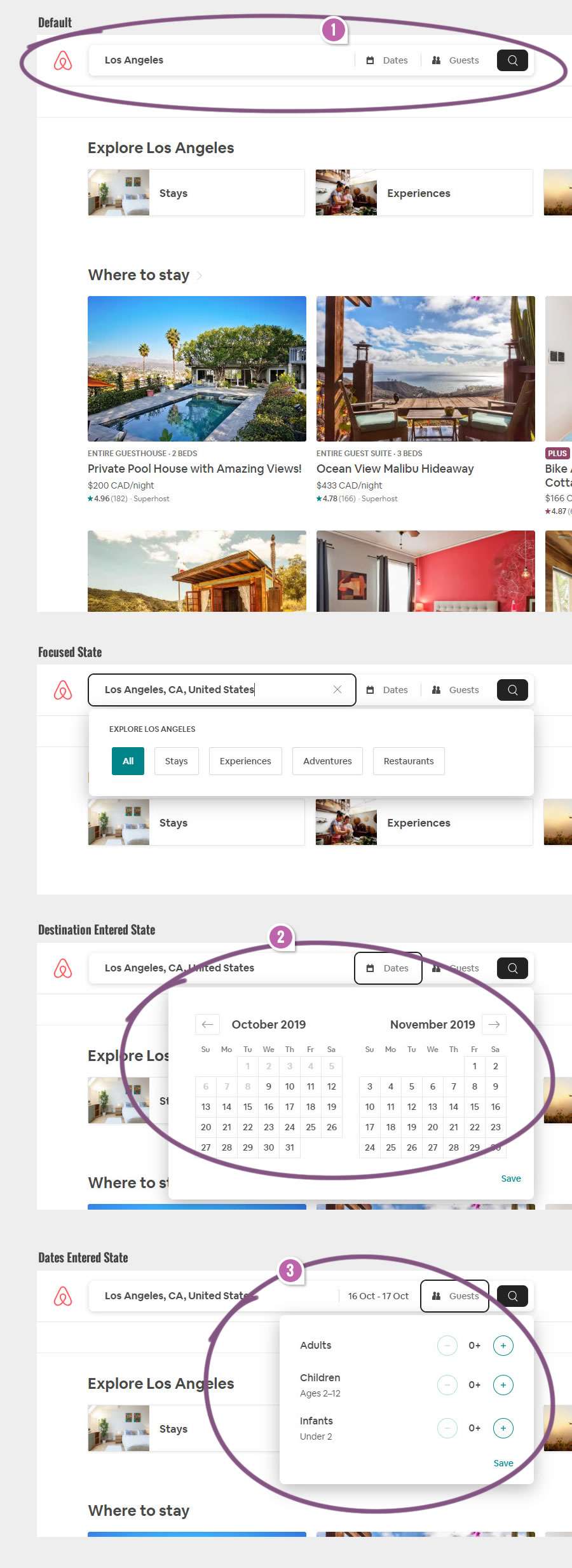The image features a webpage with a search interface centered on exploring Los Angeles. At the top of the page, within a search box, "Los Angeles" is clearly displayed alongside a purple number "1" in the top center, indicating the first step in the search process. Surrounding the search box is a distinct purple circle outline.

Below the search box, the text "Explore Los Angeles" is prominently positioned. Directly underneath this text are categories such as "Days" and "Experiences." Further down, the section titled "Where to Stay" showcases various hotel options with image thumbnails, featuring names like Kuhn, Willow, Malibu, and a "Private Pool House with Amazing View," though the text isn't entirely legible.

At the very bottom of the page, there's a weather forecast stating "Los Angeles, CA, United States." Adjacent, a navigational bar features buttons labeled "All Stays" and "Experiences," with the "All Stays" button highlighted in blue.

Further down, in another search box outlined in purple, several options and fields are visible, including "Destination," "Internal," "Destination Entered State," and "People (Adults and Children)." Specific dates "November 2019" and "October 2019" are also noted, each accompanied by the number "2" inside a purple circle and further steps marked with numbers "1," "2," and "3" highlighted in pink with white outlines.